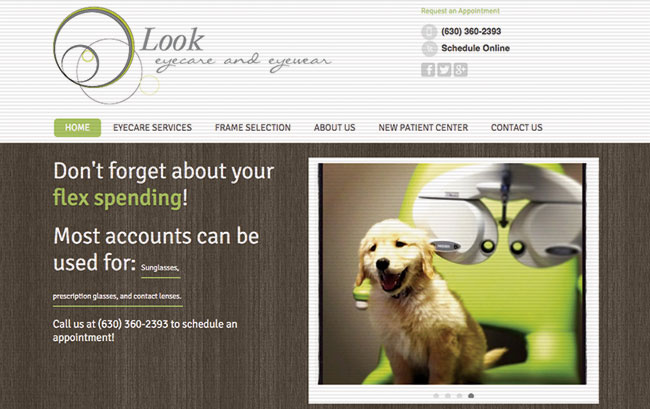At the top of the screen, there is a subtly striped gray border featuring two-tone hues of white and dark gray. The border prominently displays the text, "Look I Care and I Wear," accompanied by two circles—one in shades of green and gray and the other in just gray. To the right, there's information on how to "Request an Appointment," including a phone number (630-360-2393) and an option to schedule online. Below this, there are icons linking to Facebook, Twitter, and Google Plus.

A navigation menu spans the top, listing clickable pages: Home, Eye Care Services, Frame Selection, About Us, New Patient Center, and Contact Us. The "Home" page is highlighted with a green backdrop and white font, indicating it is the current page. Below, a reminder states, "Don't forget about your flex spending. Most accounts can be used for sunglasses, prescription glasses, and contact lenses." It encourages users to call 630-360-2393 to schedule an appointment. This section is set against a vertically oriented, faux-wood brown backdrop.

To the right of this text, there is a Polaroid-style image depicting a golden-colored dog sitting on a green chair next to an ophthalmic device used for eye examinations.